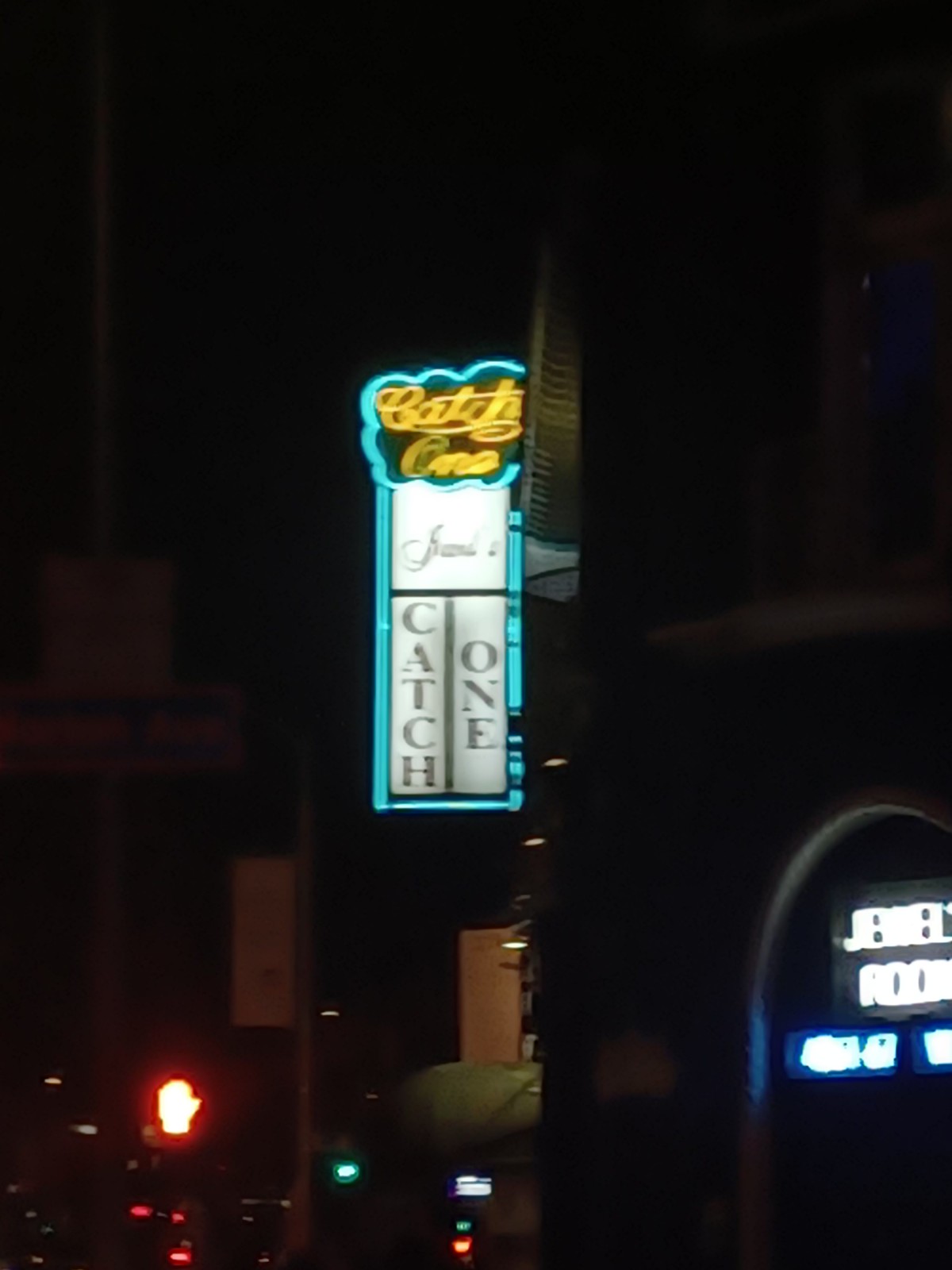This nighttime photo captures an outdoor scene with a prominent neon sign as its focal point. The sign, possibly affixed to a building, is largely rectangular with a cloud-like design at the top. It features a bright blue-turquoise neon border. The cloud-like upper section has a darker background with "Catch 1" written in yellow cursive. Below, the rectangular portion of the sign has a white background with a single horizontal and vertical line dividing it into three sections. The top section contains some unreadable text, while the bottom section prominently displays "Catch 1" in large capital letters. The background is illuminated with various lights, including an orange pedestrian signal indicating not to cross and another set of indistinct neon letters in white and light blue on the right side.